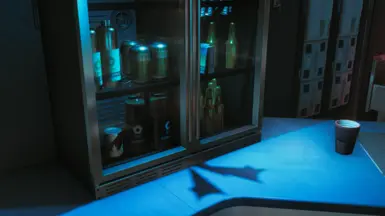The dimly-lit photograph depicts a compact, countertop refrigerator or wine cabinet, which appears suitable for storing a variety of beverages. The appliance, sleek and narrow, is situated on a blue countertop with a glass placed next to it. Behind the unit, decorative paneling adds a touch of elegance, while the area beneath the blue surface reveals a white base.

The entire scene is enveloped in dark blues and blacks, with prominent shadows accentuating the contrast. The refrigerator, designed with double glass doors, showcases its contents across four distinct shelving units, each fully stocked.

The top shelf holds two tall bottles and three standard-sized cans, likely beer. The second shelf features what appears to be a Red Bull can accompanied by two other drink containers. Midway down, the left side of the refrigerator houses champagne bottles with another can positioned nearby. The bottom shelf is lined with several upright bottles, completing the diverse collection of beverages.

This setup resembles a minibar typically found in a hotel, offering a selection of drinks for guests to enjoy.